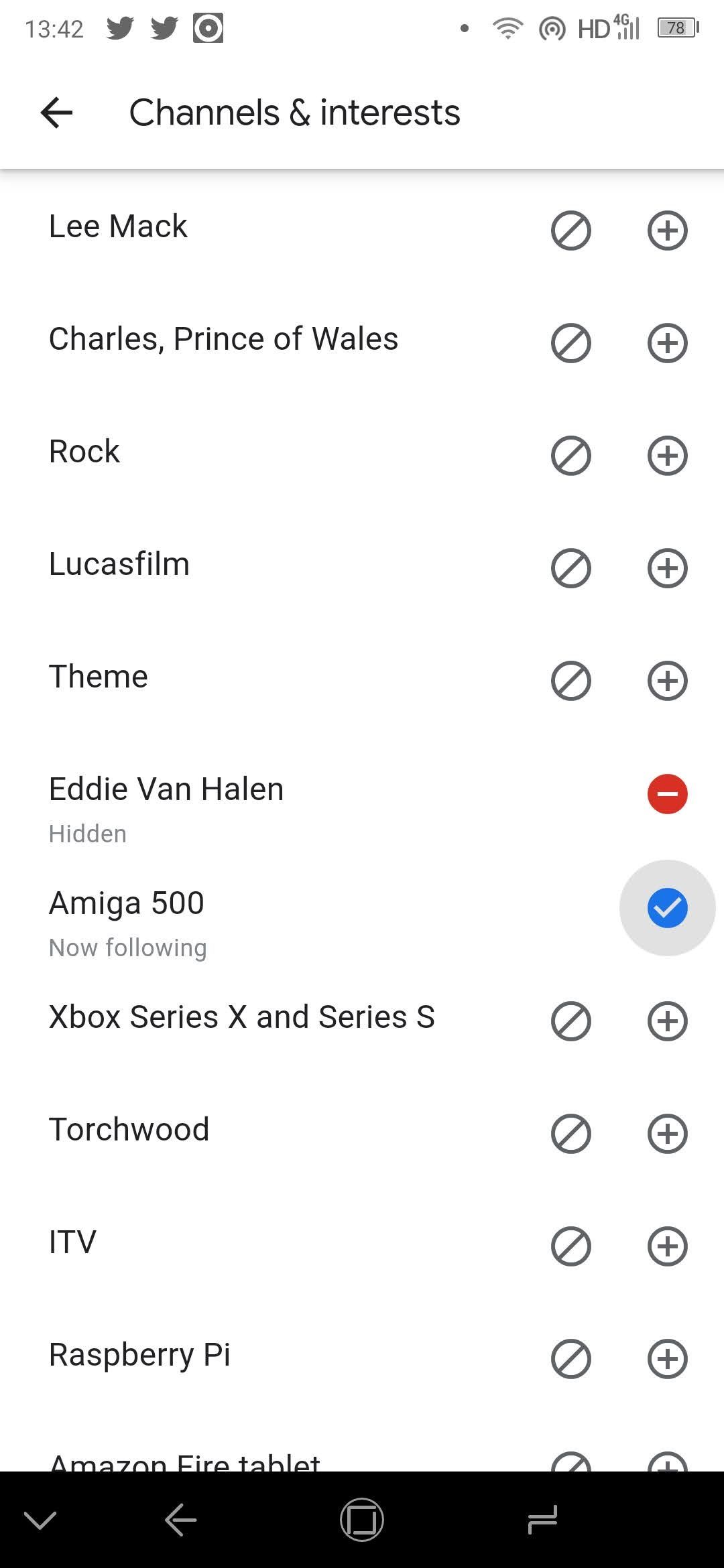**Caption:**

A detailed image captured on a smartphone screen, showcasing a white background with various interface elements. At the top, a timestamp reading "13:42" is displayed. Nearby, on the upper right, symbols indicate connectivity: Wi-Fi bars, status, HD, 4G, and a battery level at 78%. On the upper left, two Twitter bird icons and a square bullseye icon are visible.

The main content consists of a list of names aligned on the left, each accompanied by different control symbols on the right. The first entry is "Lee Mack," followed by a circle with a diagonal line and a circle with a plus sign. This pattern continues down the list: "Charles, Prince of Wales," "Rock," "Lucasfilm," "Theme," "Eddie Van Halen," "Amiga 500," "Xbox Series X and Series S," "Torchwood," "ITV," "Raspberry Pi," and "Amazon Fire Tablet." 

Distinct variations appear with "Amiga 500," marked "Not Following" and having a blue checkmark, and "Eddie Van Halen," labeled "Hidden" with a red circle and a white dash. 

At the image's bottom, a black bar features navigation icons: a down arrow, a left arrow, and two unidentified icons on the right.